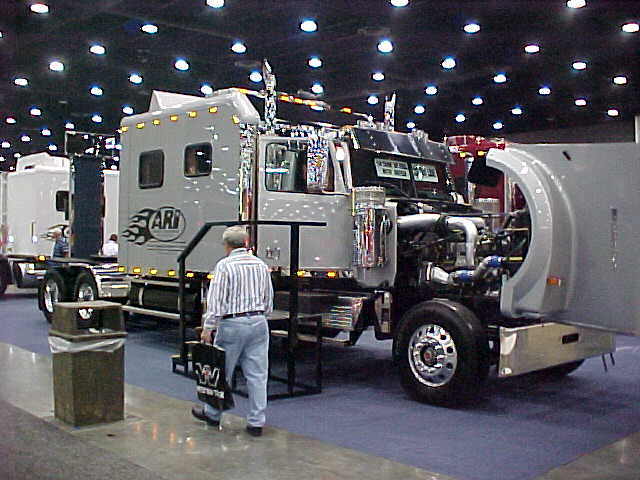The image depicts a sleek, silver tractor-trailer truck meticulously showcased inside a sophisticated showroom. The ceiling above is black, adorned with multiple spotlights that cast bright white illumination across the space. The showroom features an elegant combination of gray marble flooring and a purple rug positioned beneath the truck.

The truck, resembling a Mack model, boasts a striking appearance with extensive chrome details and black trim. It features a double sleeper cab, implying luxurious and possibly well-equipped interiors. The vehicle's hood is open, revealing a powerful, intricately designed engine with the ARI logo and a flame motif on the side. Multiple windows and several running lights adorn its structure, and there seem to be solar panels integrated into its design, reinforcing its custom-made, top-tier status.

In the foreground, a man with gray hair, dressed in a gray and white long-sleeve collared shirt and blue jeans, is captured walking past the vehicle, carrying a black bag marked with a 'W'. Beside him is a gray trash can with a white bag inside. The composition suggests that the truck might be undergoing servicing or inspection, but its grand presentation and the setting also indicate a display meant to highlight the vehicle’s premium features and exceptional build quality.